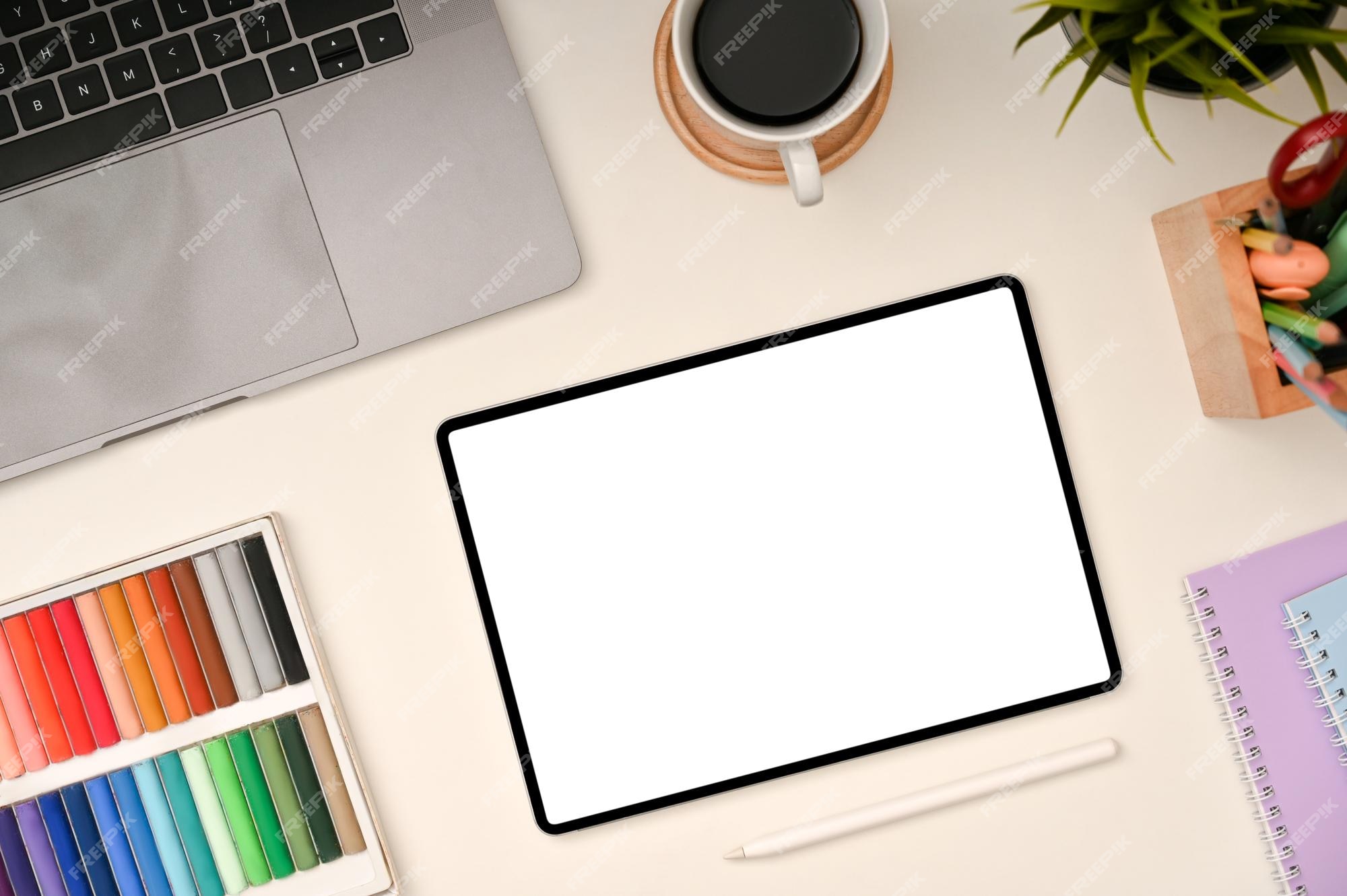This is an overhead view of a neatly organized computer desk, characterized by a recurring light gray "free pick" watermark scattered across the image. Dominating the upper left corner, there's the corner of a space gray MacBook with black keys. Centered at the top, a white coffee cup filled with black coffee sits on a circular brown wooden coaster. On the upper right, a potted plant extends its green leaves into the frame, followed just beneath by a square wooden pen holder containing pencils, red scissors, and markers. 

In the lower right corner, the edges of two spiral notebooks are visible, with the top one being light blue and the one beneath it light purple. Centrally placed, a tablet-like device with a white screen is bordered by a black rectangular frame, possibly serving as a mock-up placeholder. Below this device lies a long white pen. The lower left corner is occupied by a tray filled with colored art supplies, possibly chalk or pastel pencils, arranged in an orange, reddish, blue, and green color scheme. The entire composition is set against a creamish pink desktop that provides a soft, inviting background to this creative workspace.